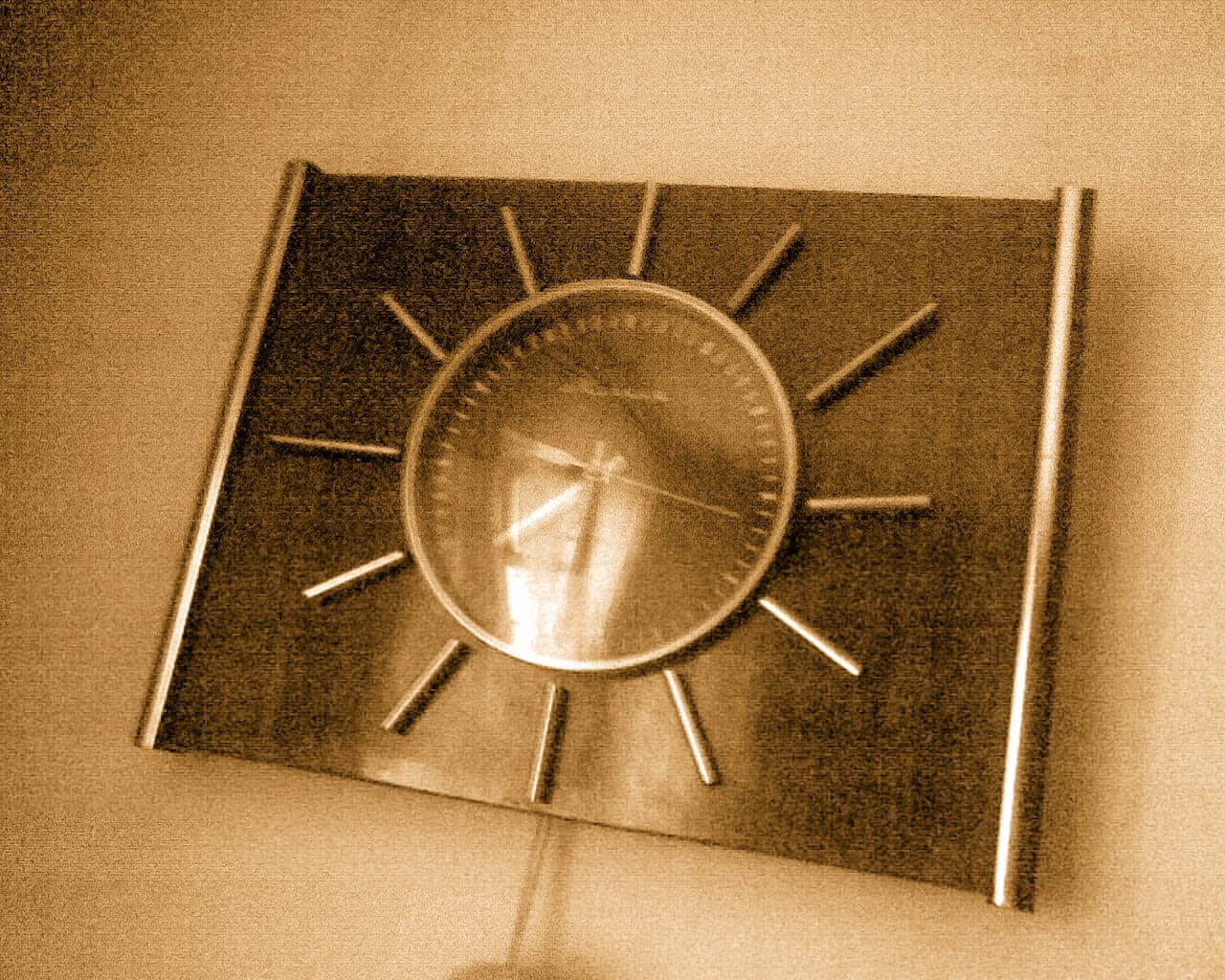A sepia-toned abstract photograph of a clock. The visually striking image features a clock with a rectangular body, upon which a dark circular clock face is mounted. Encircling this clock face are thin metal lines that add a geometric flair. The clock face itself, adorned with dashed lines, displays three distinct hands. A cord extends downward from the main body of the clock, adding to the abstract nature of the composition. Despite the super grainy texture, the photograph maintains high visual quality, enhancing its vintage charm and intricate details.